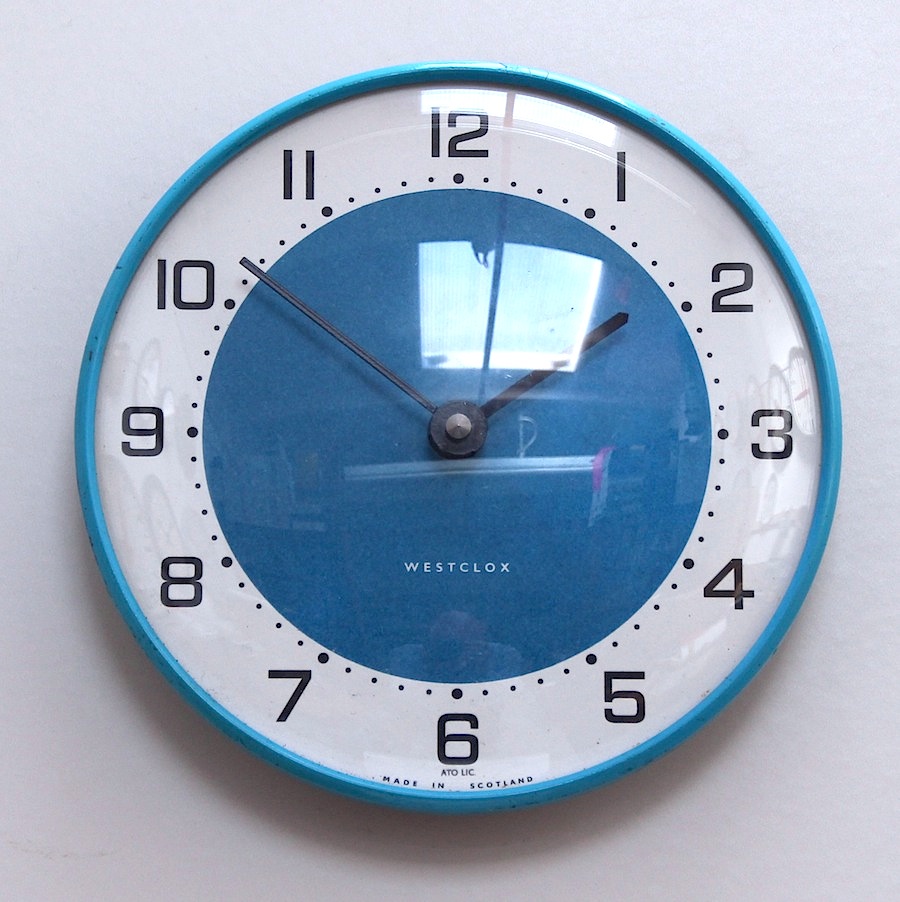Photograph of a wall-mounted clock displaying the time as 1:52. The clock's center features the brand name "WESTCLOX" in white lettering. The clock face has a dark blue background, with black numbering set against a light blue border. The black hour and minute hands are covered by a clear, reflective surface—possibly glass or plastic. This surface reflects light, showing an image of a white window near the top of the clock, just below the numeral 12. The clock is placed on a white wall.